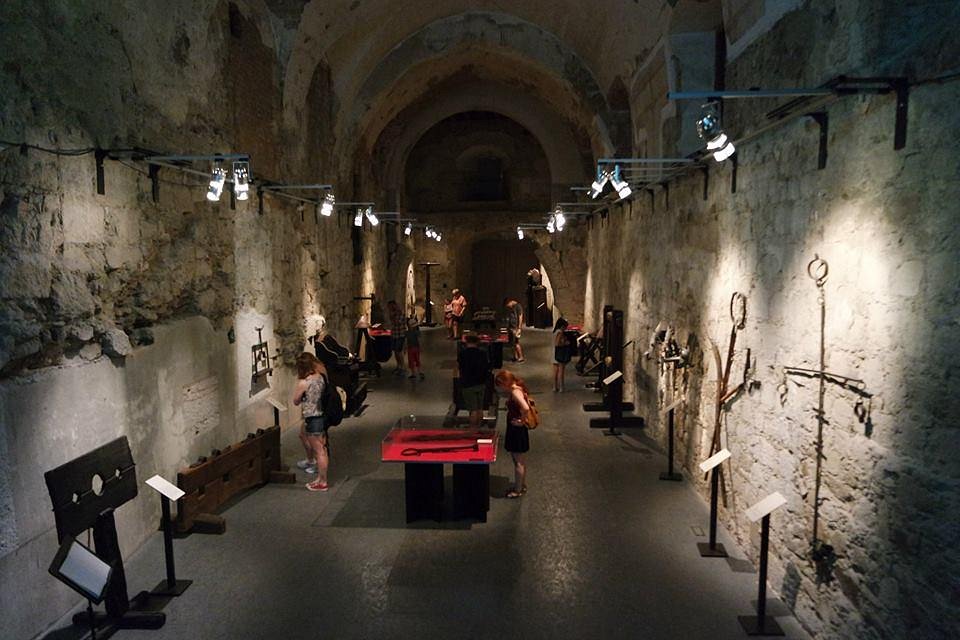The image depicts an underground or dimly lit museum exhibit inside what appears to be an ancient stone fortress, tunnel, or cathedral-like space with high ceilings. The walls are lined with various artifacts that resemble ancient relics or perhaps torture devices, each illuminated by strategically placed lighting fixtures. Some of these items, such as swords, are displayed on tables covered in red tablecloths, while the walls boast items that could be whips or similar implements. A notable scene centers around a lady examining one of these tables intently. Information podiums stand before each wall display, providing details about the museum-quality items. Visitors are dispersed throughout the space, engaging deeply with the exhibits both on the walls and in the center of the hallway, thoughtfully reading the podiums and observing the relics. The atmosphere is one of historical intrigue, amplified by the aged, stone construction and the somewhat eerie ambiance.